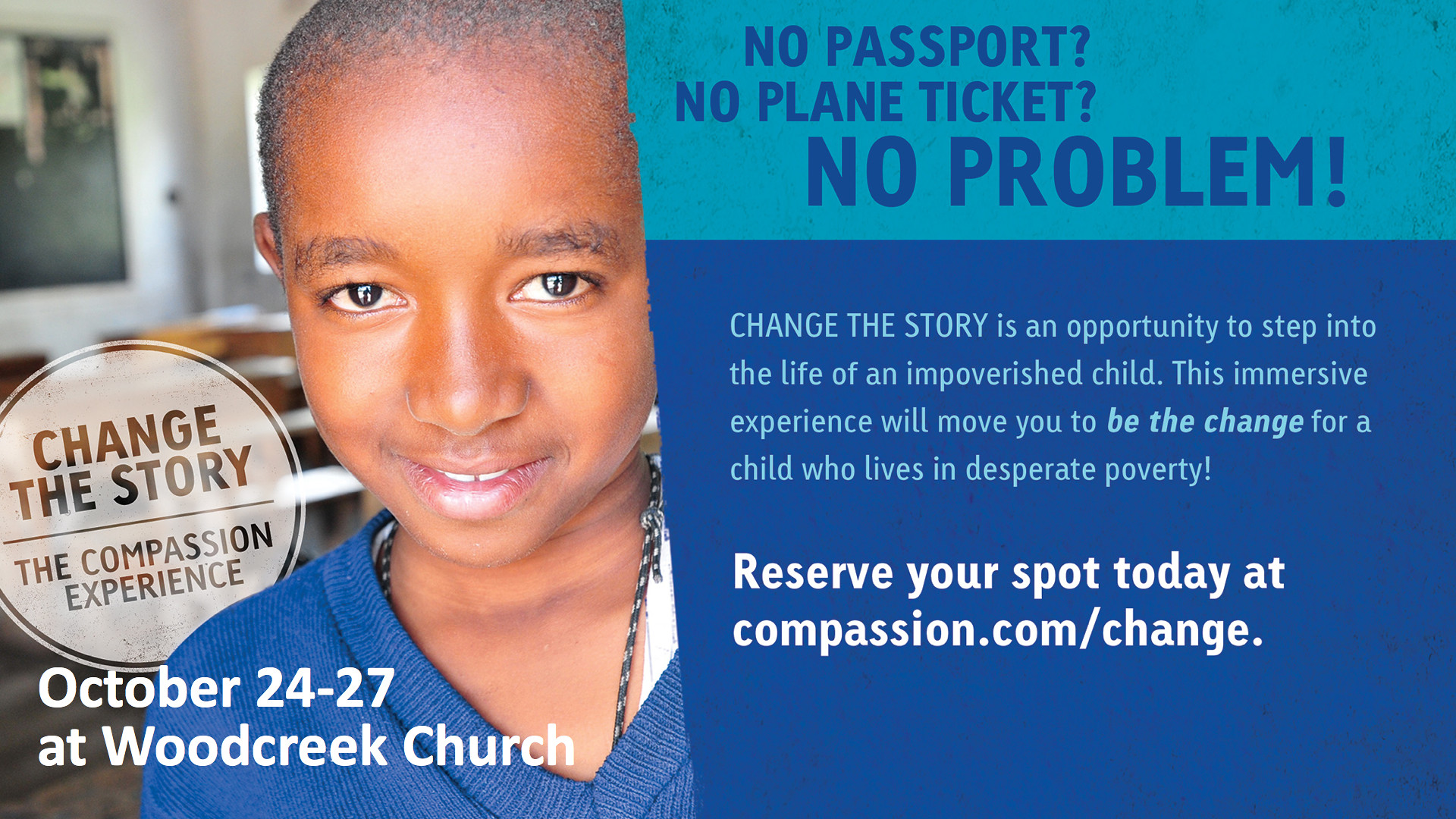The promotional flyer features a color image of a young, dark-skinned boy with a small smile, gazing directly into the camera. The photo, which takes up the left half of the flyer, shows the boy inside what appears to be a classroom, with tables and chairs visible in the background. He is wearing a simple chain and a blue shirt, adding to the casual and relatable atmosphere of the scene.

To the right of the image, bold text in various shades of blue and white details the event: "Change the Story: The Compassion Experience, October 24 to 27 at Wood Creek Church." Further down, it reads, "No passport, no plane ticket, no problem." This immersive event provides an impactful opportunity to step into the life of an impoverished child, aiming to inspire attendees to become agents of change for children living in desperate poverty. Interested participants are encouraged to reserve their spot at Compassion.com/change.

The flyer effectively uses a minimalist color palette of blues, white, and a few earthy tones to draw attention to the poignant message and the hopeful expression on the child's face, compelling viewers to engage with the cause.